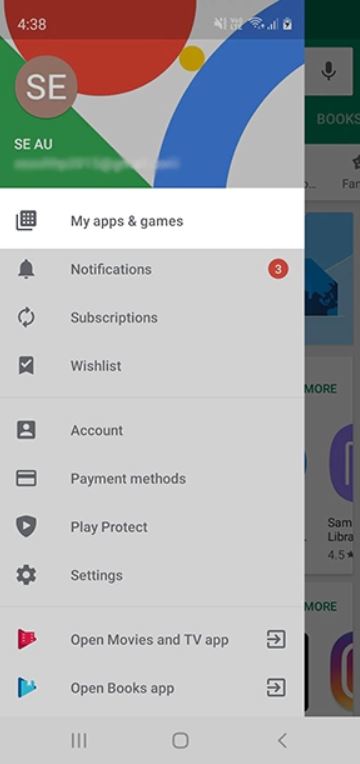The image appears to be a screenshot of a mobile app interface, possibly from a Google Play Store menu, displaying various sections and options. At the top of the screen, there is a gray rectangle with a green triangle in the lower left corner. Positioned above this is a brownish circle inscribed with "SE". Behind this, a portion of a red circle containing the number "438" is visible, next to which lies a yellow circle. An angled blue line is also present, accompanied by some white markings beside it. 

Further down, there is a square with white dots inside it and an adjacent line. Below this segment, the text "My Apps and Games" is clearly displayed. To the right, a bell icon labeled "Notifications" is shown with a red circle indicating the number "3". Below these options are additional items including:

- Two circular arrows forming a loop labeled "Subscriptions".
- A bookmark icon with a checkmark captioned "Wishlist".
- A gray square containing a person symbol titled "Account".
- A credit card icon labeled "Payment Methods".
- A shield with an arrow pointing right titled "Play Protect".
- A gear icon labeled "Settings".

Further down, there is a red, indeterminate icon that reads "Open Movies and TV App". Alongside it is a gray-outlined square with an arrow pointing right. Below these, a blue symbol resembling the red one reads "Open Books App", accompanied by another square with an arrow pointing right. 

At the bottom of the screen, three closely aligned lines and a gray-outlined square with an arrow pointing left are visible. In the background, particularly on the far right side, multiple elements are grayed out, including:

- A gray box overlaying other items
- A green element
- A microphone icon
- Some text
- A blue element
- Additional text
- A purple element
- A multicolored item